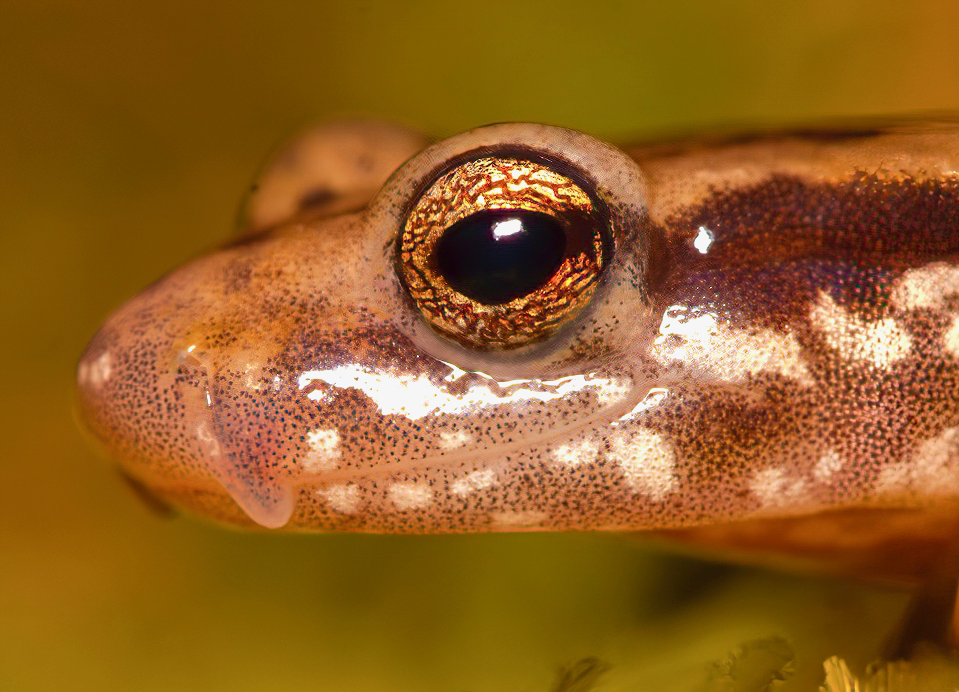This full-color, square photograph, likely taken outdoors, portrays a professionally staged nature shot focusing on the close-up head of a reptilian creature, either a snake or a lizard, although some details suggest it might be a frog. The creature's large, black eyeball is accentuated with striking orange bands, and the eye appears somewhat bloodshot. Reflective skin, possibly due to a camera flash, has a shiny texture with a surface that may contain some slime, particularly around the mouth. The muzzle is moist, with visible slime dripping from the upper to lower lip. The creature's skin showcases a dynamic palette of white splotches and black splotches against an orange or light brown backdrop. Behind its eye lies a distinct black band followed by a dark brown one. The end of the head curves slightly. The blurred, greenish hue of the background provides minimal contextual clues, keeping full focus on the intricate, detailed features of the creature itself. The other eye can be seen, slightly out of focus, in the background.